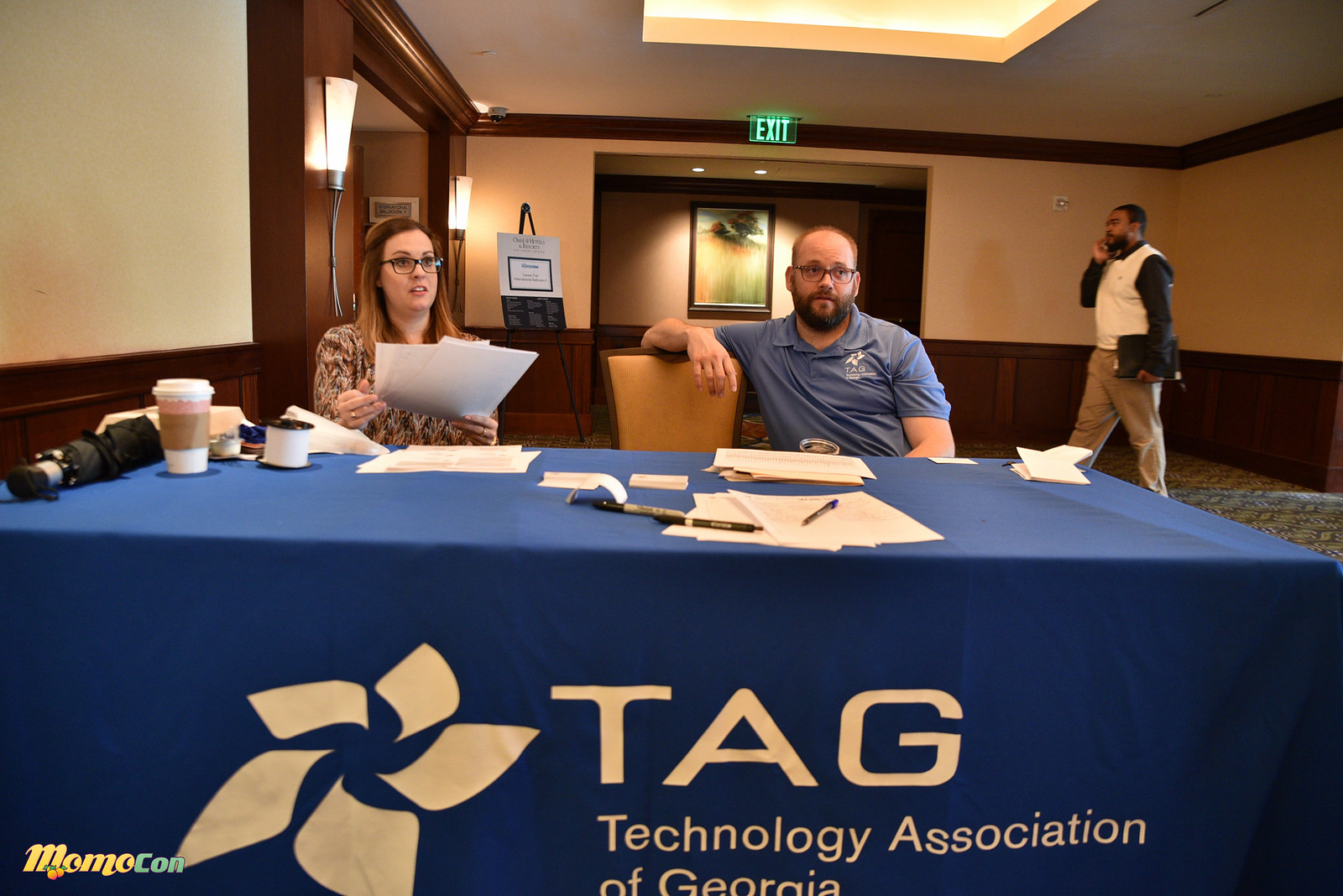The image shows a room, possibly at a conference or hotel, with three people prominently featured. In the foreground, a rectangular table is covered with a blue cloth that has the logo "TAG: Technology Association of Georgia" along with a twisted star design on the left side. The table is cluttered with coffee cups, papers, an umbrella, and pens. 

Seated at the table, on the left side, is a woman with long blonde hair wearing black glasses. She is dressed in an orange and white small top jacket. She holds some papers in her hand and appears to be speaking while looking toward the front right. To her right sits a man with a thin brown beard and mustache, wearing a blue polo shirt with the TAG logo. He has brown hair, glasses, and his arm rests on the back of a nearby brown chair, also looking in the same direction as the woman.

In the background, a man with short brown hair, possibly African American, walks past while talking on a phone and carrying a satchel. He is dressed in a black long-sleeved shirt and a white vest. The room itself has a cream-colored upper wall, wood grain lower wall, and wooden framing around doorways. There are green exit signs and a recessed ceiling with multiple lights. On the wall behind, there is a portrait of trees and flowers in a field.